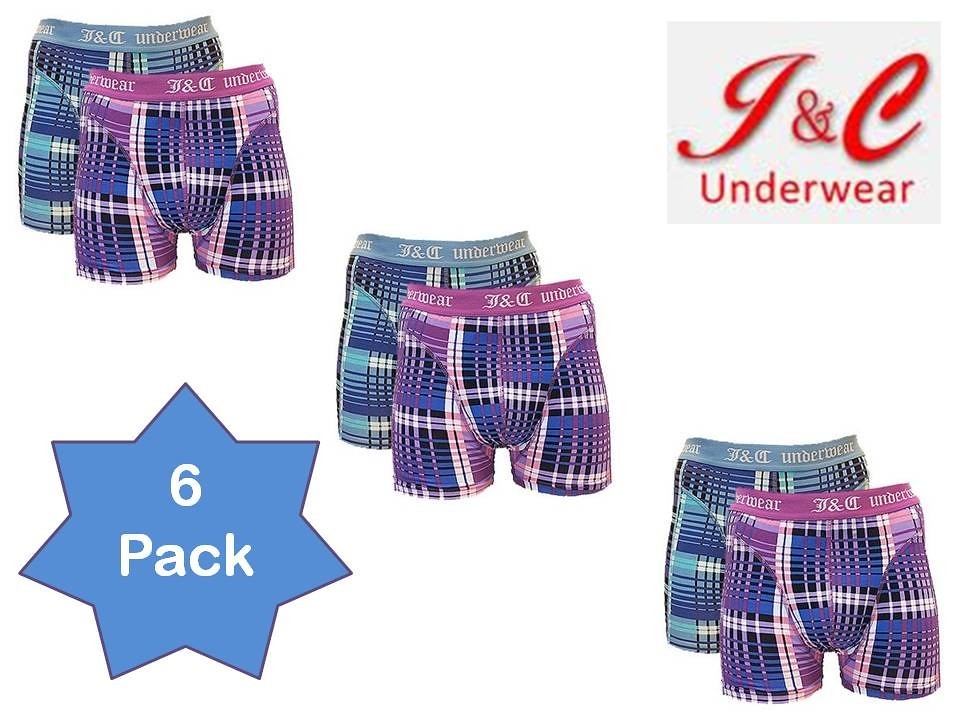This advertisement features a six-pack of men's boxer briefs by J&C Underwear. The packaging prominently displays a white rectangle with "J&C Underwear" written in red letters and a blue star-shaped sticker indicating "six-pack" in white letters. Each six-pack contains two distinct plaid designs, shown in sets of two. One design includes a violet-purple color scheme with black, white, and purple elements, featuring a matching elastic waistband that says "J&C Underwear" in white. The other design showcases a combination of slate blue, black, and white plaid with a corresponding slate blue waistband, also branded with "J&C Underwear" in white. All pairs reach mid-thigh and are described as snug-fitting, highlighting a mix of colorful plaid patterns with teal, navy, black, and various shades of blue and purple.